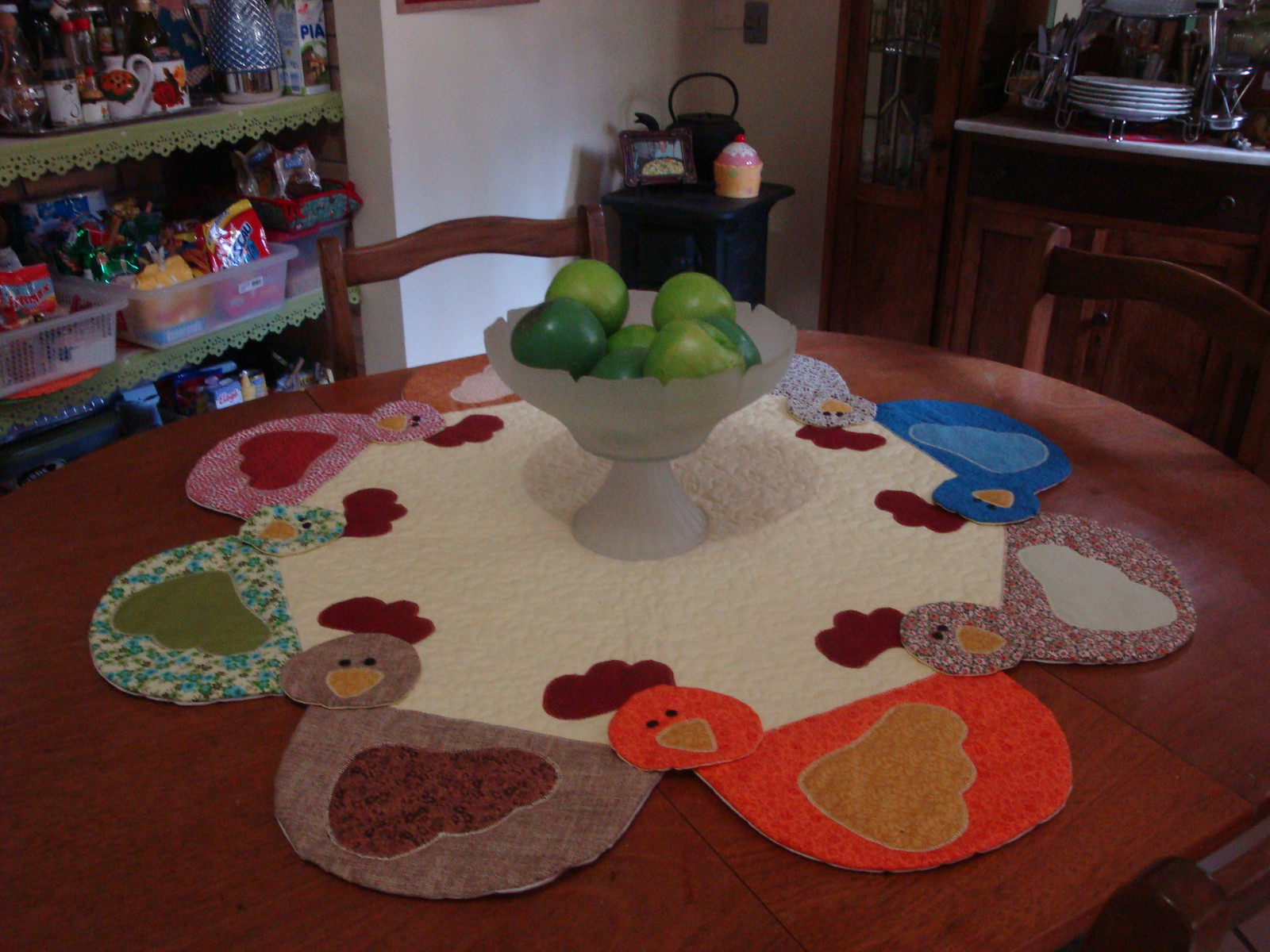The photograph is an indoor color scene taken in low light, depicting a cozy kitchen environment. The focal point centers on a round dark brown wooden table, which is topped with a large, textured, embroidered placemat featuring minimalistic cartoon depictions of hens or chickens in a variety of colors, including orange, brown, and light blue, around its circumference. The centerpiece on the placemat is a frosted, bell-shaped glass bowl with an intricate, ridged stem, filled with several light green apples that slightly overflow above the bowl's lip. This bowl casts a soft shadow on the placemat. 

In the background, along the left-hand wall, are shelves crammed with plastic bins filled with food, toys, and kitchen utensils, displaying a sense of cluttered warmth. A white wall behind these shelves is discernible, with what appears to be a wooden or cast iron stove laden with a couple of objects. To the right side of the image, there is a china cabinet showcasing an array of dishes and plates. The image, slightly out of focus and dimly lit, captures a homey, well-used kitchen space, complete with two chairs tucked around the table, emphasizing the lived-in feel.